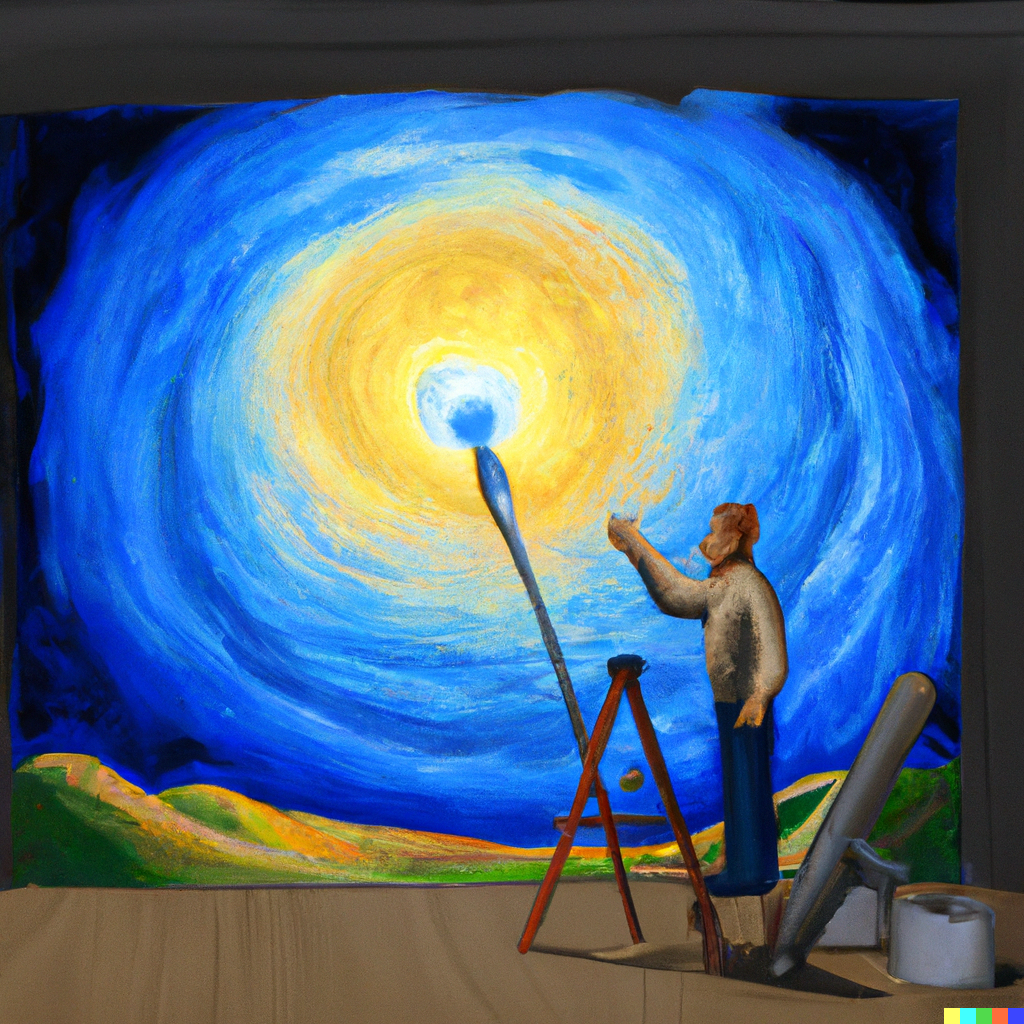The image showcases an artistic interpretation of an artist at work. It presents a square canvas with no definable border or background, featuring a multi-color palette with hints of digital enhancement. At the center of the image stands the artist, wearing a beige sweater and jeans, depicted with a simple, non-detailed face in profile. The artist stands on a brown wooden stage, possibly a box or platform, with a large canvas in front of them.

The artwork on the canvas is dominated by a central blue dot, surrounded by concentric swirls of white, yellow, lighter blue, and darker blue, invoking the impression of a wormhole. Interestingly, a large paintbrush leans against the canvas, extending all the way down to the floor, though the artist is not holding it. The artist's right arm is extended towards the blue center, almost pointing with a sense of purpose.

In the very lower right-hand corner of the piece, several colored squares are scattered, seemingly unrelated to the main composition. Under the artist, a white paper roll extends outward, and beneath them is a brown canvas. Additional elements include abstract representations of mountains in green and yellow hues at the bottom of the painting. The overall scene is a vibrant and dynamic display of colors, including light green, light yellow, orange, dark yellow, deep red or maroon, gray, and silver.